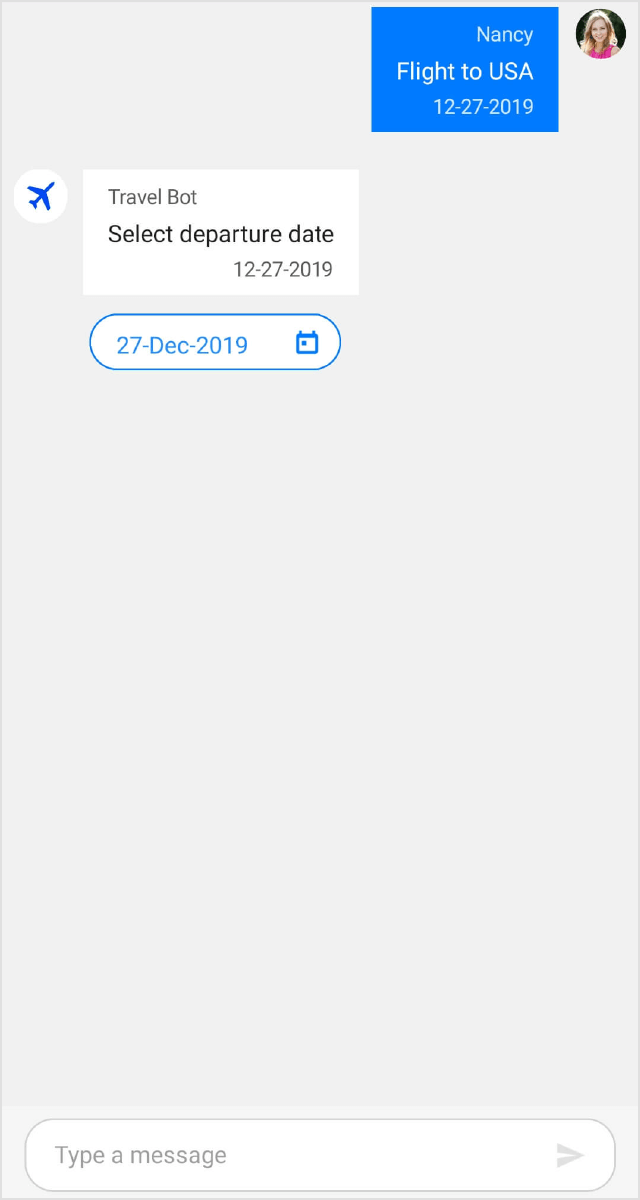This is a detailed screenshot of a chat interaction. The background of the screenshot is white, and in the top right corner, there is a circular profile picture with a black background. Inside this circle is an image of a white girl with shoulder-length blonde hair, wearing a pink shirt.

The girl, identified as Nancy, has sent a message that appears in a blue text box. Her message reads "N-A-N-C-Y" followed by "F-L-I-G-H-T-T-O-U-S-A" and beneath that is the date "12.27.2019."

Below Nancy's message, there is a response from the left side, where the profile picture is a white circle containing an airplane icon. The responder is identified as "travel bot," and their message is housed in a white text box. The message from the travel bot reads: "Select departure date 12.27.2019," followed by "27/D-E-C/2019." The date seems to be formatted differently to give clarity to the user.